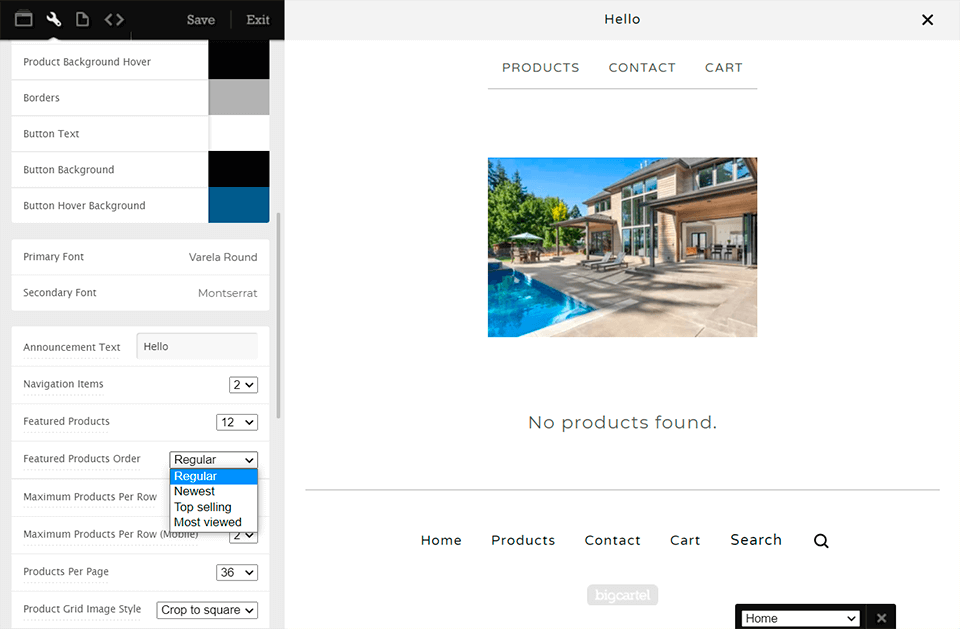This image displays a website interface, characterized by a layout approximately 30% wider than it is tall. The interface features a vertical navigation column on the left, occupying about one-third of the screen from top to bottom. This navigation column is topped by a black bar containing several icons: a horizontal rectangle, a wrench, a page, and two arrows pointing left and right. Additionally, in the upper right corner of this section, there are "Save" and "Exit" buttons.

The navigation column includes various selectable white bars with associated options on their right side. The options visible include settings such as "Product Background Hover" set to black, "Borders" set to gray, "Button Text" in white, "Button Background" in black, and "Button Hover Background" in medium blue. The primary font is indicated as "Varelia Round" and the secondary font as "Monoscript." Below these settings, another section offers additional customization options.

On the right-hand side of the interface, a light gray bar spans the top, occupying the remaining two-thirds of the screen's width. This bar centers the word "Hello" in its text. Beneath this, the background transitions to white and presents navigation options labeled "Products," "Contact," and "Cart." An image of an outdoor pool is displayed in this section, followed by the text "No products found."